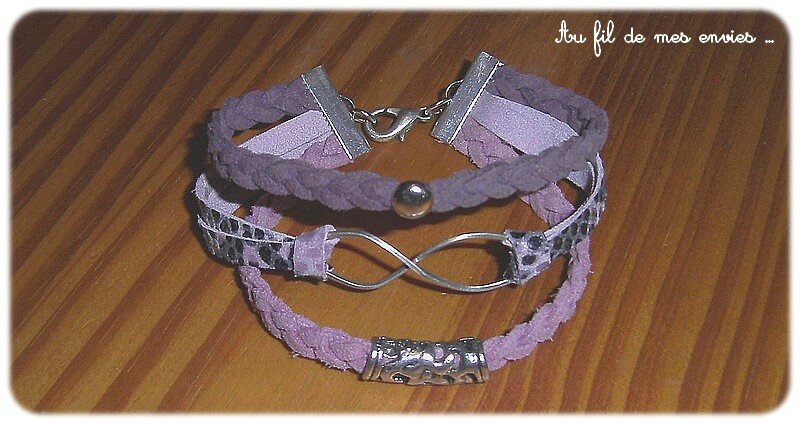In the center of a wooden table lies a detailed, triple-layered purple bracelet composed of three distinct parts, each connected to a silver bar at the back with a secure clasp. The bottom layer showcases a lavender braided leather strap adorned with a silver cuff featuring intricate designs. The middle bracelet stands out with a silvery tone and a prominent purple shine, highlighted by an infinity hoop at the front. The top layer is a deeper purple braid, ornamented with a small, round silver circle at its center. The entire bracelet ensemble, resting horizontally on the table, appears positioned for a product photograph against a backdrop of angled wood grain. Surrounding the bracelet are fragments of text, reading "O, Phil, D, Mess," and other partial letters, adding an element of mystery to the setting.